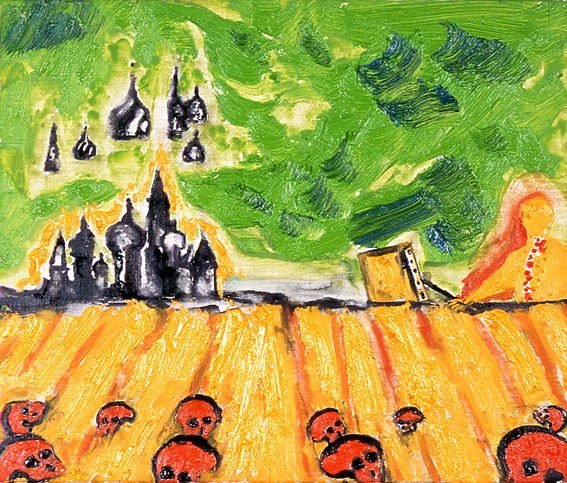This square painting, reminiscent of a crayon or cartoon style, features distinct segments with vibrant colors and detailed elements. At the very bottom, red skulls with black eyes and noses are scattered on an orange field, possibly resembling soil or hay. There are around 10 of these skulls, outlined in black, lying on an orange ground with vertical red lines.

The midsection of the artwork is divided by a black line, separating the bottom from a castle-like structure on the left. This castle, depicted in gray, white, and black, has several towers and steeples, and its upper parts are mirrored as floating images in the sky above.

On the right side of the middle section, an outline of a person with long red hair in orange can be seen, though only the head and shoulders are discernible. The upper portion of the painting is primarily green with blue smears, especially on the right side and upper left corner, suggesting a lush, Van Gogh-inspired landscape with hills and additional architectural elements.

Overall, the painting conveys a surreal scene where the organic and architectural coexist in a dreamy, almost whimsical manner.